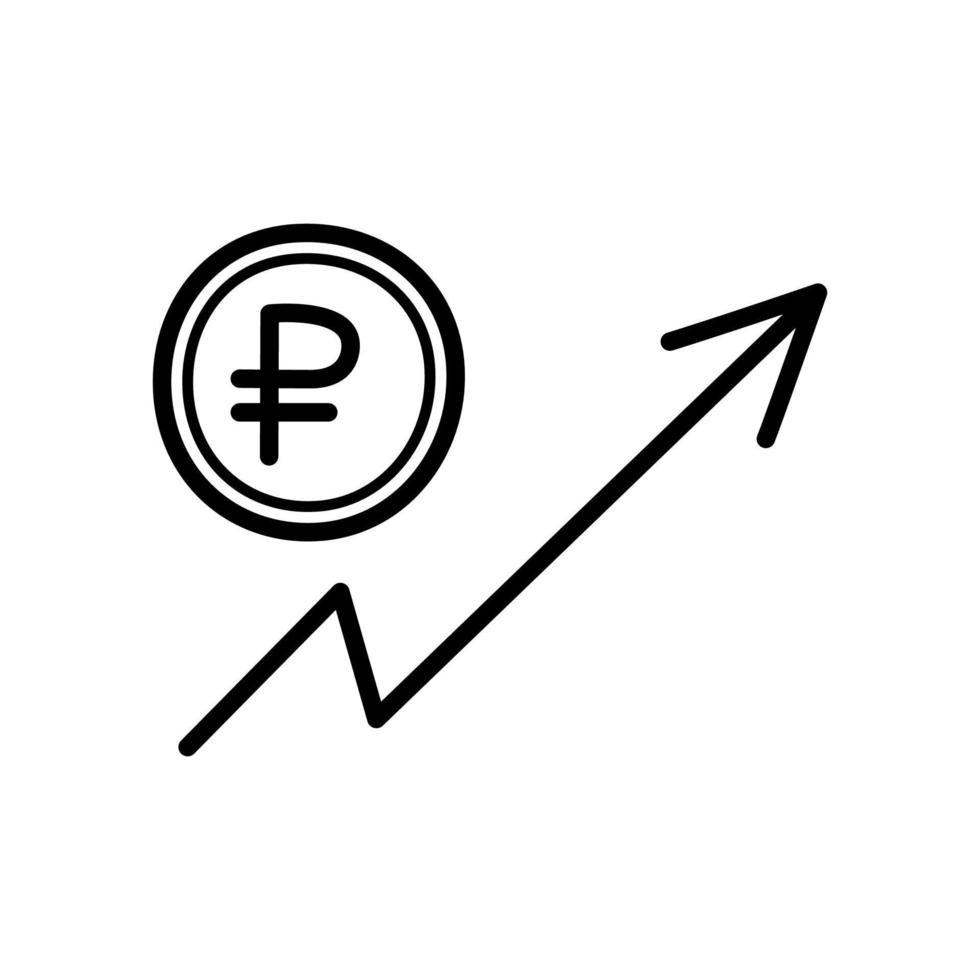The image depicts two distinct black symbols on a plain white background. The first, located in the upper left portion of the image, is a double-ringed circle with a thicker outer circle and a thinner inner circle, both encircling a white center. Within this center is a stylized "P" character, featuring a horizontal line that crosses just beneath the loop of the "P". The second symbol is a jagged arrow that starts at the bottom left corner, rises slightly, dips down momentarily, and then ascends sharply to the top right, resembling a lightning bolt or an erratic line in a financial graph. The arrow ends with a conventional arrowhead.